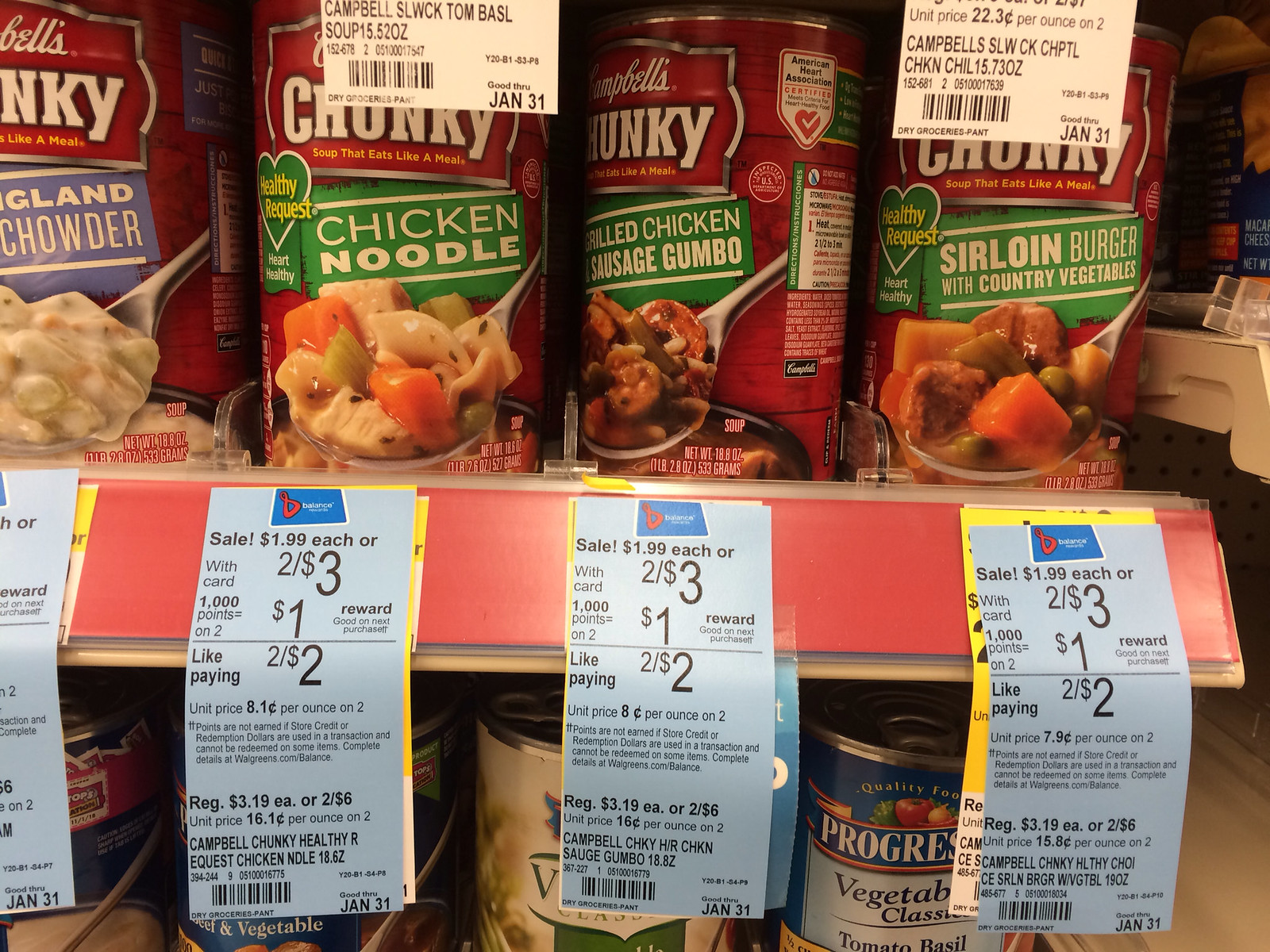A detailed display of the soup aisle showcases a variety of options, with clearly marked price tags at the bottom. Prominently featured at the top, Chicken Noodle Soup stands out with its distinct label, followed by other flavorful choices such as Grilled Chicken Sausage Gumbo and Sirloin Burger with Country Vegetables. The lower section houses additional soup varieties, all neatly organized. Adding a pop of color, a red bin is visible at the bottom, possibly for promotions or special items. The arrangement is tidy, ensuring easy visibility and selection for shoppers.